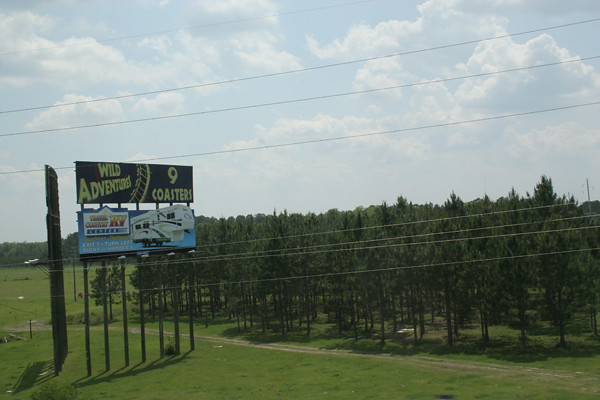A vibrant outdoor photo captures the roadside scene dominated by a towering two-story banner. On the top half, a striking black banner with bold yellow text proudly advertises "Wild Adventures: Nine Coasters." Below, a blue banner showcases an RV dealership, featuring a white RV image, although the text is unreadable. This large billboard is mounted on six sturdy wooden poles, standing prominently beside a rustic dirt trail that weaves through the scene. Power lines stretch across the foreground, connecting to a weathered wooden utility pole. Beyond the trail, an orderly array of trees, possibly part of a tree farm or a deliberately planted grove, extends into the distance, offering a blend of nature and human enterprise in a single frame.